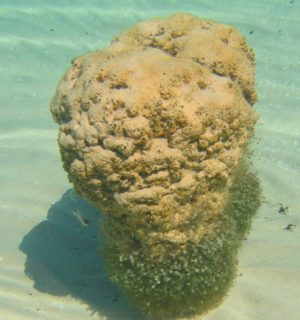This underwater photograph captures a large, tan-colored coral reef or rock formation submerged in clear, greenish-blue water. The focal point is a rugged, bulbous mass with a surface resembling human brain folds, featuring various shadings of khaki and light brown. Its top half appears rock-like, rough, and clumpy, while the bottom half, edging the pale and rippled seafloor, is surrounded by vibrant green seaweed or moss. Scattered around this enigmatic underwater object are small, gray fish, adding a subtle motion to the scene. The entire formation casts a shadow on the sandy seabed, emphasizing its three-dimensionality. The overall image conveys a peaceful, underwater landscape dominated by this intriguing coral structure.